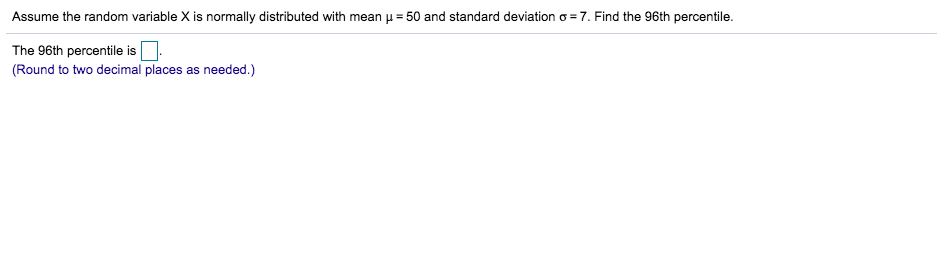A very wide screenshot captures a mathematical instruction. The text directs the user to "assume the random variable X is normally distributed with mean (μ) = 50 and standard deviation (σ) = 7. Find the 96th percentile." This is displayed on a white background, implying a digital or online question, possibly from an AI or search engine interface.

Below the question is a blue underline, suggesting an input field or emphasis on the next section, followed by the phrase "The 96th percentile is a square," with a note in parentheses advising the user to "round to two decimal places as needed." The text is rendered in small black letters, with the only color being the blue underline and the emphasized square and rounding instructions. The layout is exceptionally wide, stretching end-to-end across the page, with no additional content beneath it.